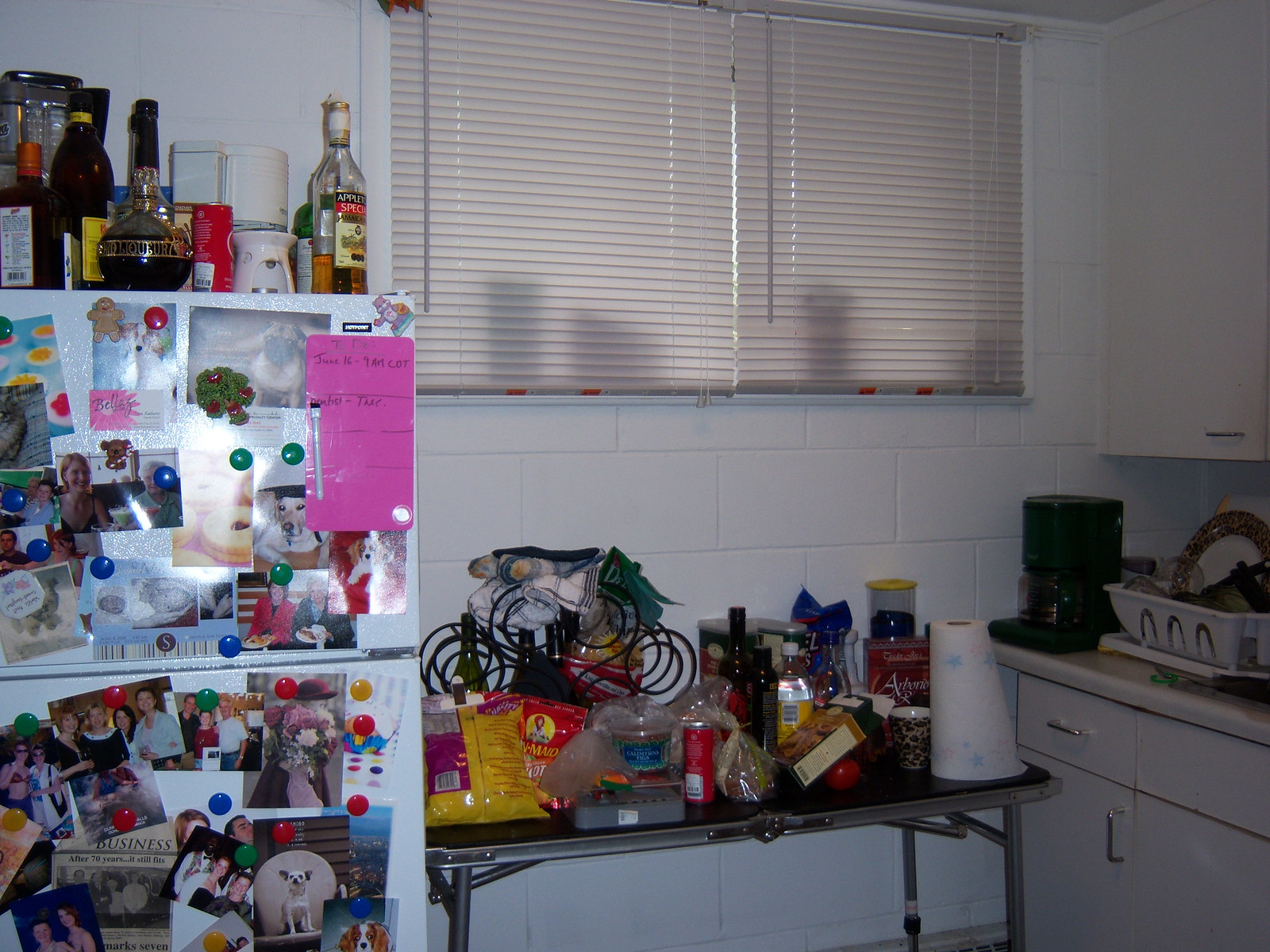An image captures an extremely messy kitchen scene dominated by white and off-white tones. The back wall is covered in large white tiles with precise white grout lines. Above a counter, there are two large windows with cream-colored, horizontal shades drawn down, casting faint shadows. The shades are suspended on a rod that matches their color, blending seamlessly with their surroundings.

To the left of the windows stands a white refrigerator, its surface almost entirely obscured by an assortment of photographs, papers, and colorful magnets in red, green, yellow, and blue hues. Atop the refrigerator are several bottles, prominently featuring a clear glass liquor bottle containing brown liquid and adorned with a beige label with red and black accents. Next to it is a distinctive Chambord bottle, oval-shaped and clear with a black top and a gold metallic band around its center, filled with dark purple liquid. Additionally, a dark brown Kahlua bottle with a yellow label, another dark bottle with a red cap, and an unidentifiable bottle clutter the space.

In the foreground, a long, foldable metal table, cluttered with a roll of white paper towels with blue floral prints, multiple food boxes, and packages, extends across the scene. A wire shelf, seemingly designated for wine storage, peeks from the back.

To the right, a section of white cabinetry and shelving houses more kitchen essentials. A white strainer with dishes, a black electric coffee maker, and pristine white cabinets complete the disorganized yet detailed tableau of everyday life captured in this busy kitchen.